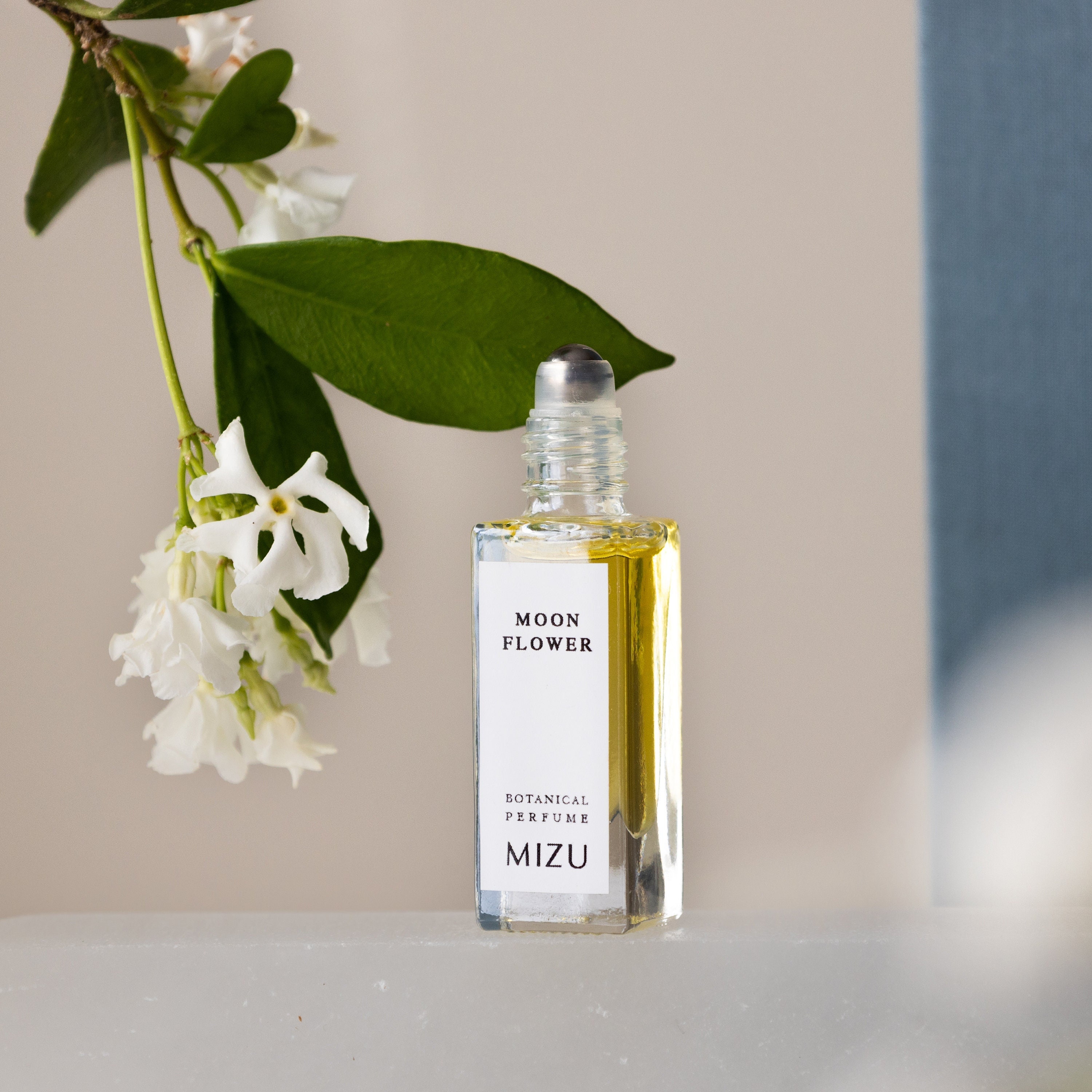The photograph showcases a clear glass perfume bottle set on a white table. The background features a predominantly white wall, with a thin blue strip descending about two-thirds down the right side. The bottle contains a yellowish liquid and sports a white label with black lettering. The label reads "Moonflower" at the top and "Botanical Perfume, MIZU" at the bottom. The bottle is a roll-on type, topped with a silver metal ball, and the cap is removed, revealing the ball applicator. Notably, a green stem with white trumpet-shaped flowers and yellow centers extends from the top left corner towards the bottle. The image also has a slight white smudge at the bottom right, possibly from the camera lens.